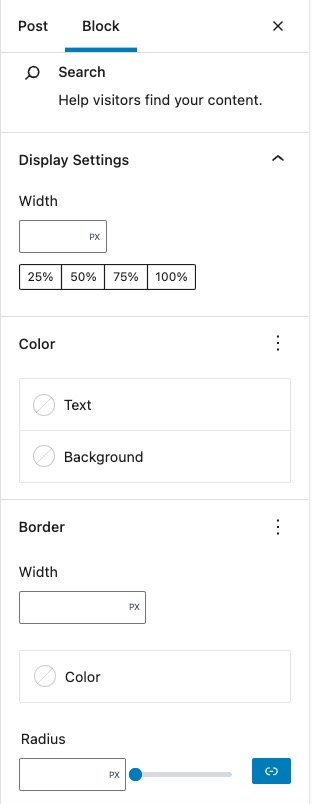The image showcases settings from a phone app or a programming interface, presented in a portrait orientation and framed by thin gray borders on the top and bottom. The overall layout is approximately three times taller than it is wide, juxtaposed on a primarily white background with black text.

At the very top of the image, there's a narrow horizontal header housing two options: "Post" and "Block," with an 'X' situated on the right side. The "Block" option is underlined in blue, indicating it is selected.

Beneath this header, a segmented box contains a search icon depicted as a magnifying glass, labeled "Search," with a supplementary note saying, "help visitors find your content."

Following this, another box occupies about half the page height, labeled "Display Settings." To its right is an upward caret (^). This section details:
- "Width," with an adjacent empty input box labeled "PX."
- Four selectable boxes with percentages ranging from 25% to 100%.

Further down, under a header "Color," are two boxes designated for "Text" and "Background" colors, each indicated with grayed-out circles containing diagonal lines.

The final segment, titled "Border," appears in the top left of the last box. It includes:
- "Width" with an accompanying "PX" input.
- "Color" selection area.
- "Radius" with another "PX" input box below it.

A small blue scroll tab and a blue button are situated within this section, adding to the comprehensive configurability of the settings.